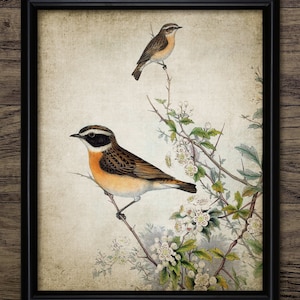The image showcases a meticulously detailed painting or drawing set on a medium brown wooden surface, possibly a countertop. At its center, the artwork is encased in a sleek black frame, standing out against a background that transitions from white to an off-white hue, creating an aged paper or canvas effect. The bottom right of the painting is adorned with a network of branches, extending upward both diagonally and vertically. The branches are rendered in shades of brown and are dotted with delicate green leaves and pristine white flowers. Perched on one of the branches in the foreground is a bird with a rich blend of brown wings, a brown head, an orange chest, and striking black and white facial stripes. Its beak and feet are a stark black. Behind this bird, another similar bird is depicted on a further branch. This secondary bird shares the same color palette, though its black facial markings and orange chest are more subdued. The intricate details of both birds, the branches, and the surrounding elements create a harmonious and lifelike scene, capturing a moment of natural beauty.